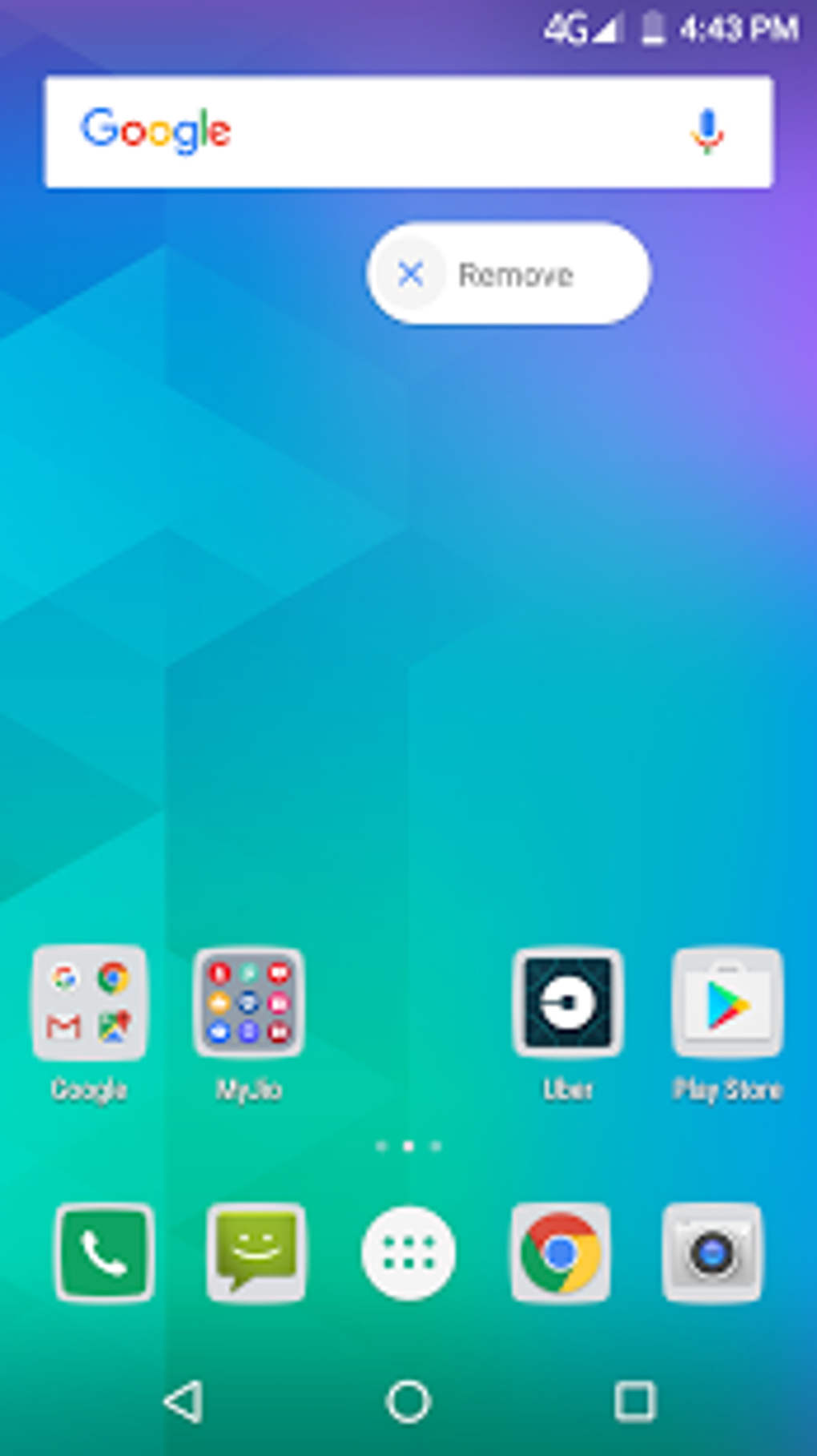The image showcases the home screen of a smartphone, specifically highlighting its Google integration and layout. At the very top, it features a Google search bar where users can type queries or use the microphone icon for voice search. The header also displays essential information including a 4G network indicator, Wi-Fi signal strength, battery life, and the current time, which is 4:43 PM. Just below the search bar is an 'X' button allowing users to dismiss the search functionality if desired. The search bar is elongated, horizontally stretched, and white, giving it an oval appearance.

Beneath the search bar, the screen is segmented into a series of app icons organized into categories. The top row is dedicated to Google applications; it includes four icons arranged from left to right: Google Search, Google Chrome, Gmail, and Google Maps. Below this, there's a somewhat blurry box containing nine additional icons, followed by standalone icons for Uber and the Google Play Store.

The next section of icons, starting again from left to right, includes a Phone app, an emoji icon with three green dots representing messaging, another Google Chrome icon, and a Camera app. At the very bottom of the screen lie the navigation buttons: a triangle for 'back', a circle for the 'home' button, and a square for accessing recent apps.